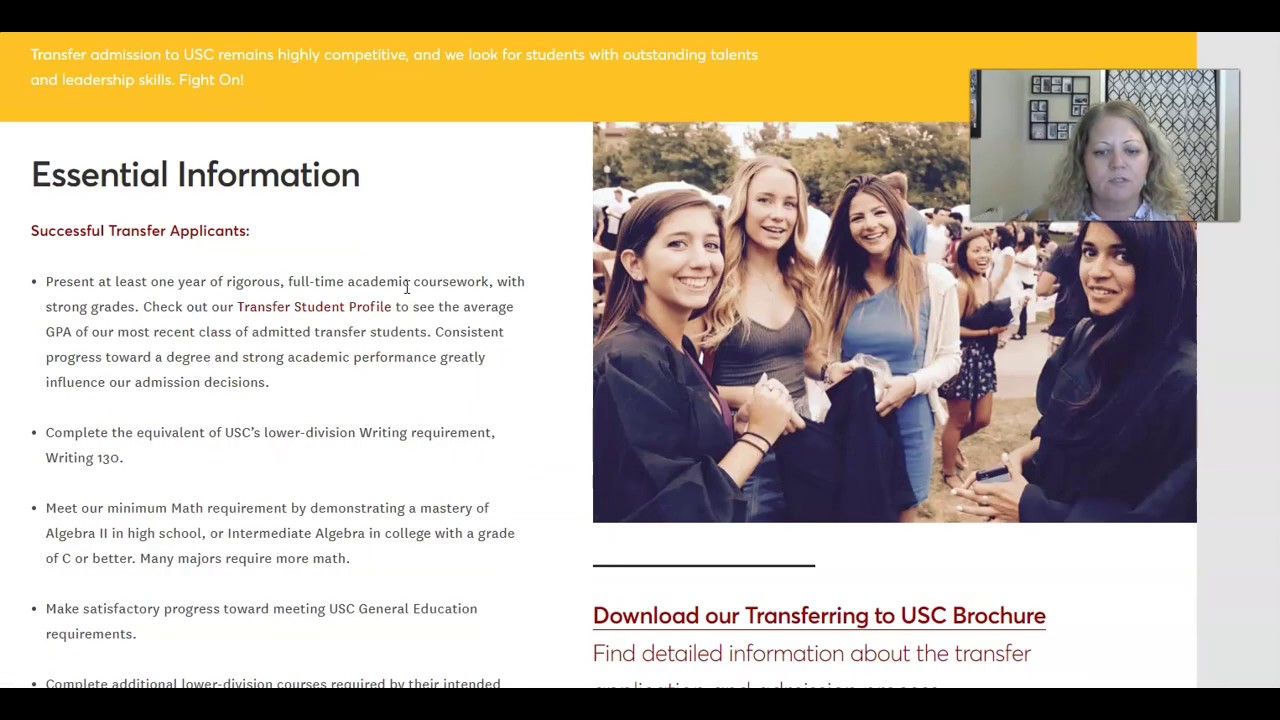This image is a screenshot from a website. At the very top, there is a thin black bar, followed by a yellow bar with white text that reads: "Transferring Admissions to USC remains highly competitive and we look for students with outstanding talents and leadership skills." Below the yellow bar, there is another thin black bar. The main body of the page is labeled "Essential Information" in a bold heading. Following this, the text discusses "Successful transfer applicants" and lists four key points:

1. The first bullet point is written as a full paragraph.
2. The subsequent three bullet points are shorter paragraphs.

On the right side of the page, there is a photograph featuring women standing outside.